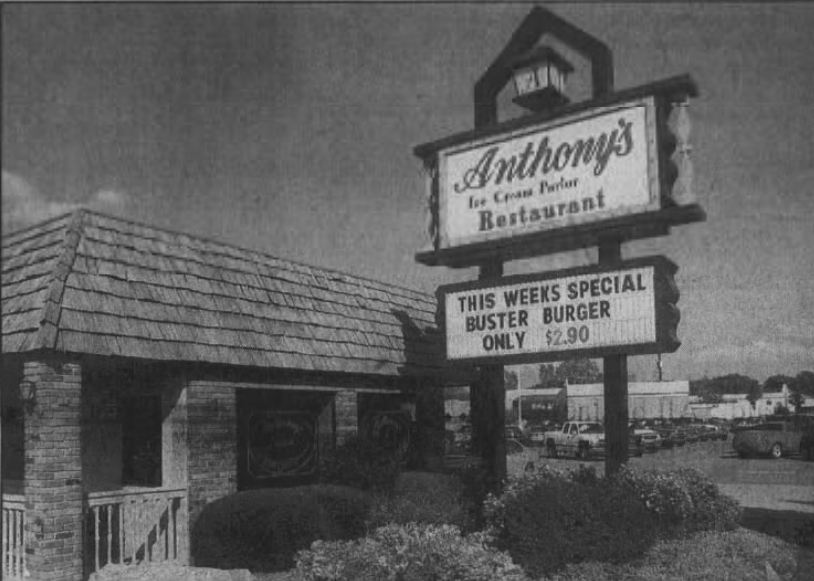This horizontal black-and-white photograph captures the exterior of Anthony's Ice Cream Parlor Restaurant. Prominently featured in the foreground is a large business sign with an overhead lamp. The sign reads in cursive, "Anthony's Ice Cream Parlor," with the word "Restaurant" in standard text below it. Beneath this, a changeable letter board announces this week's special: "Buster Burger, Only $2.90." 

The one-story building to the left of the sign boasts a classic design with wooden shingles and a mansard roof, accented by two large front windows and a set of columns at each corner. A brick facade with a front railing adds to the old-fashioned charm of the establishment. 

In the background, to the right of the sign, a bustling parking lot filled with various cars and trucks suggests a modern setting, despite the retro pricing on the sign. The presence of numerous vehicles hints at the restaurant's location in a busy or possibly industrial area where workers frequently dine. Landscape bushes are visible below the sign, contributing to the summery atmosphere, as indicated by the foliage.